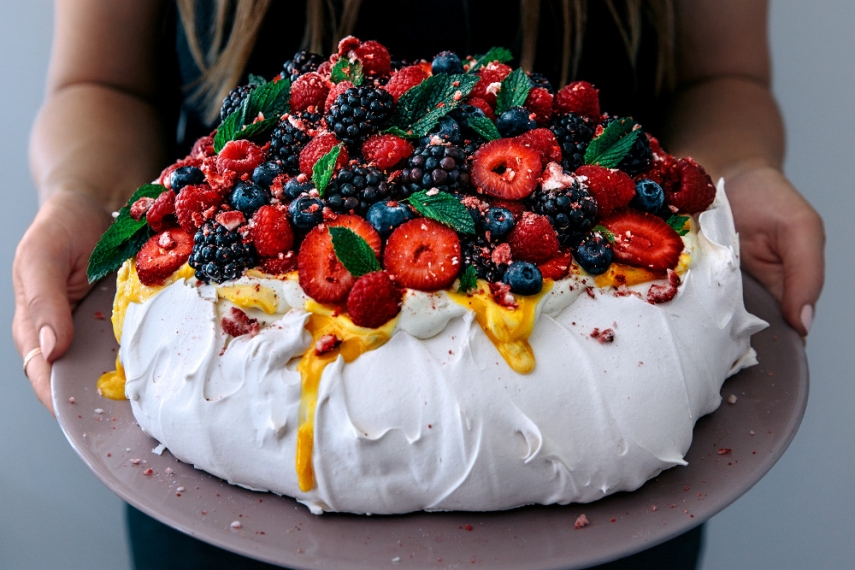The image features a woman with a bronzy-brown skin complexion and long blonde hair, extending a homemade fruit-covered cake in front of her. The cake sits on a light purple dish and presents a rustic, rounded mound with sloped sides, rather than the smooth, uniform shape typical of traditional cakes. The cake is generously coated with white icing that cascades down its uneven sides, and a golden yellow drizzle, resembling an egg yolk or honey, glimmers near the top. The summit of this confection is piled high with a vibrant assortment of fresh berries—strawberries, raspberries, blackberries, and blueberries—accentuated by sprigs of green mint leaves. The woman is only partially visible from the arms and midsection due to the angle of the shot, with the main focus being on the elaborately adorned cake.